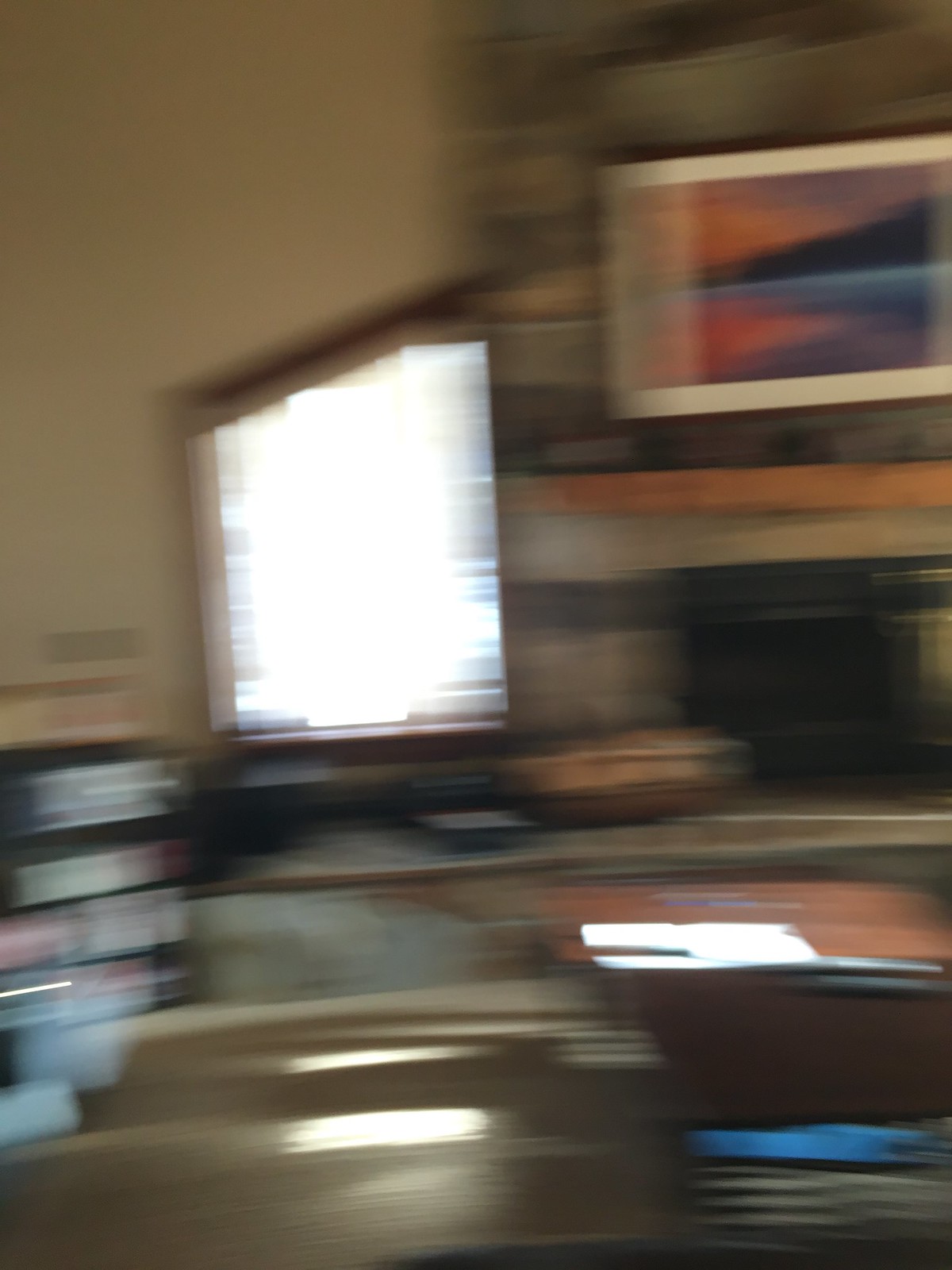The photograph depicts a blurry image of a cozy indoor living space that appears to be a living room or den. Dominating the right-hand side is a stone fireplace with a wooden mantle. Above this mantle hangs a rectangular picture frame containing an image of a lake and mountains, possibly at sunset, showcasing hues of orange and pink. Surrounding the fireplace, the walls are white. To the left of the fireplace is a large, irregularly shaped picture window with a slanted top, revealing a bright, overexposed outdoor scene. 

In the foreground, there appears to be a wooden table with a shallow wooden bowl on top and what looks like a black-framed computer monitor tilted to the left. Beside the table, there’s a sheet of white paper and what could be black and white books or objects. Visible further towards the left are another table and a shelving unit. On the ground, there seems to be a carpet. Additionally, there is a couch closer to where the picture is being taken. Despite the blurriness of the image, the elements suggest a rustic and homely living area.